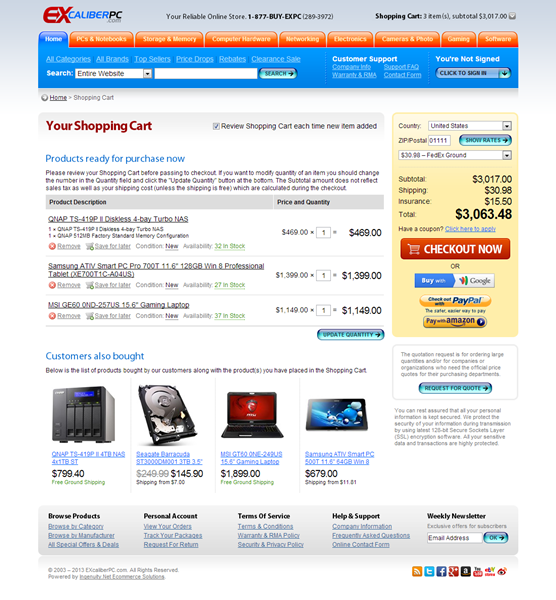This image is a screenshot of a website with a sophisticated grey and white gradient background. The background starts with a dark grey hue at the top, transitions to white in the center, and fades back to dark grey at the bottom. Positioned at the top left corner, the website's logo prominently features "EX" in large red font, followed by "Caliber" in smaller blue font, and "PC" in black font. Directly underneath "PC," the domain ".com" is displayed in black.

To the right of the logo, in black font, the text reads: "Your Reliable Online Store," followed by the customer service number "1-877-BY-EXPC," with "(2893972)" indicated in parenthesis. Adjacent to this, also in black font, it states "Shopping Cart," detailing "3 items," with a subtotal of "$3,017," accompanied by a shopping cart icon.

Below this header, a series of navigational buttons allow users to explore different sections of the site. The tabs include "Home," "PC and Notebooks," "Storage and Memory," "Computer Hardware," "Networking," "Electronics," "Camera and Photo," "Gaming," and "Software." Each tab is highlighted in red, except for the "Home" tab, which is blue, signifying that it is currently selected. Beneath this selected tab, an additional blue bar has expanded to indicate its activation.